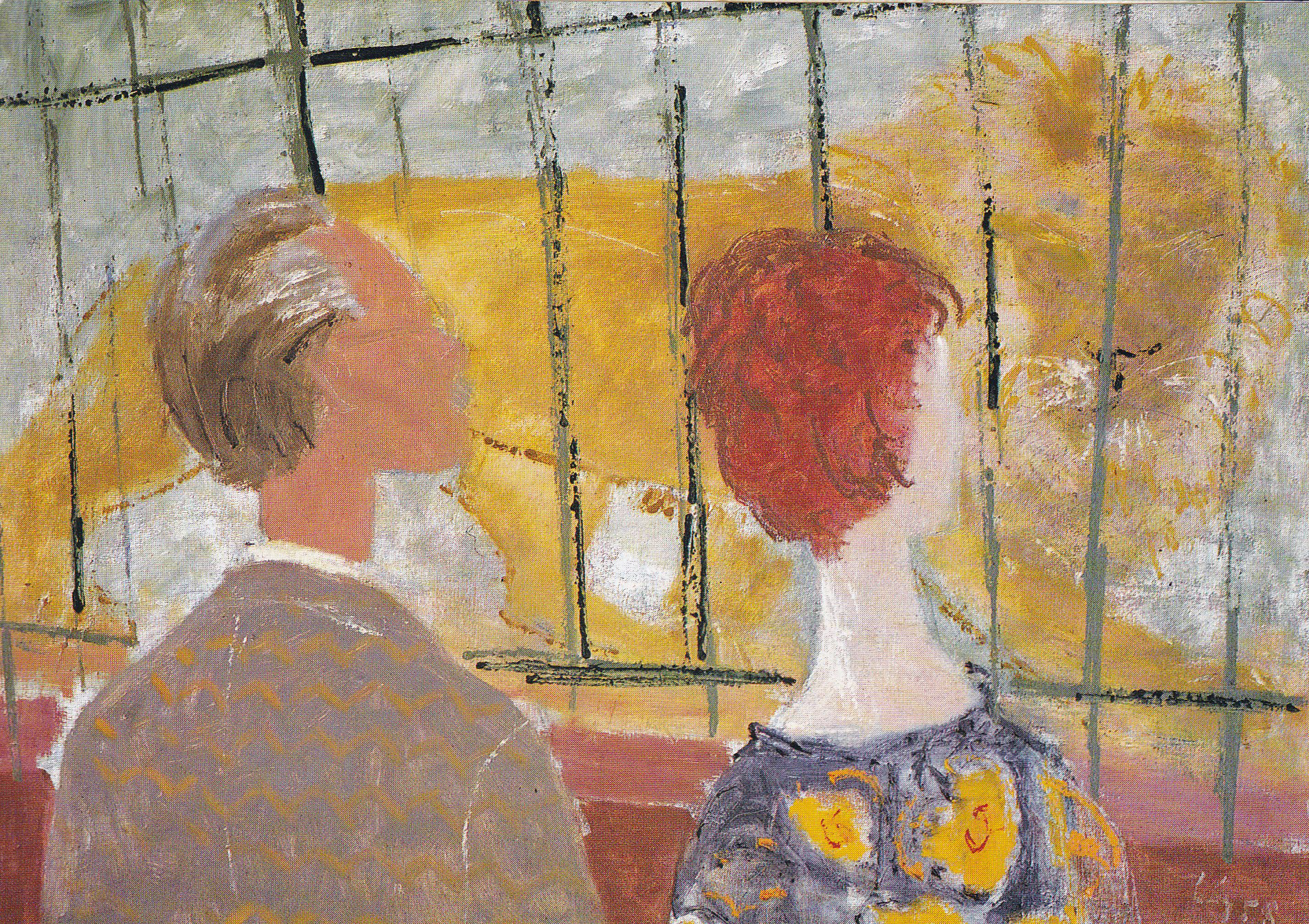This is an intricate painting portraying a couple observing a lion behind a cage. On the left stands a middle-aged man with a mix of dark brown and gray hair, accented by a mustache and round glasses. He is dressed in a distinct suit featuring a gray base with a yellow pattern. To his right, a porcelain-skinned woman with striking red-orange hair is captured in a blue gown adorned with yellow and red elements. The gown has a unique design that wraps around her neck. Both figures are focused on the lion, which is golden with hints of white in its mane. The lion resides behind a series of green slats and both diagonal and horizontal black bars atop a brick wall approximately four feet high. The background suggests a zoo setting, adding context to the scene. In the forefront, there appears to be the artist's signature done in white, positioned in the bottom right corner.